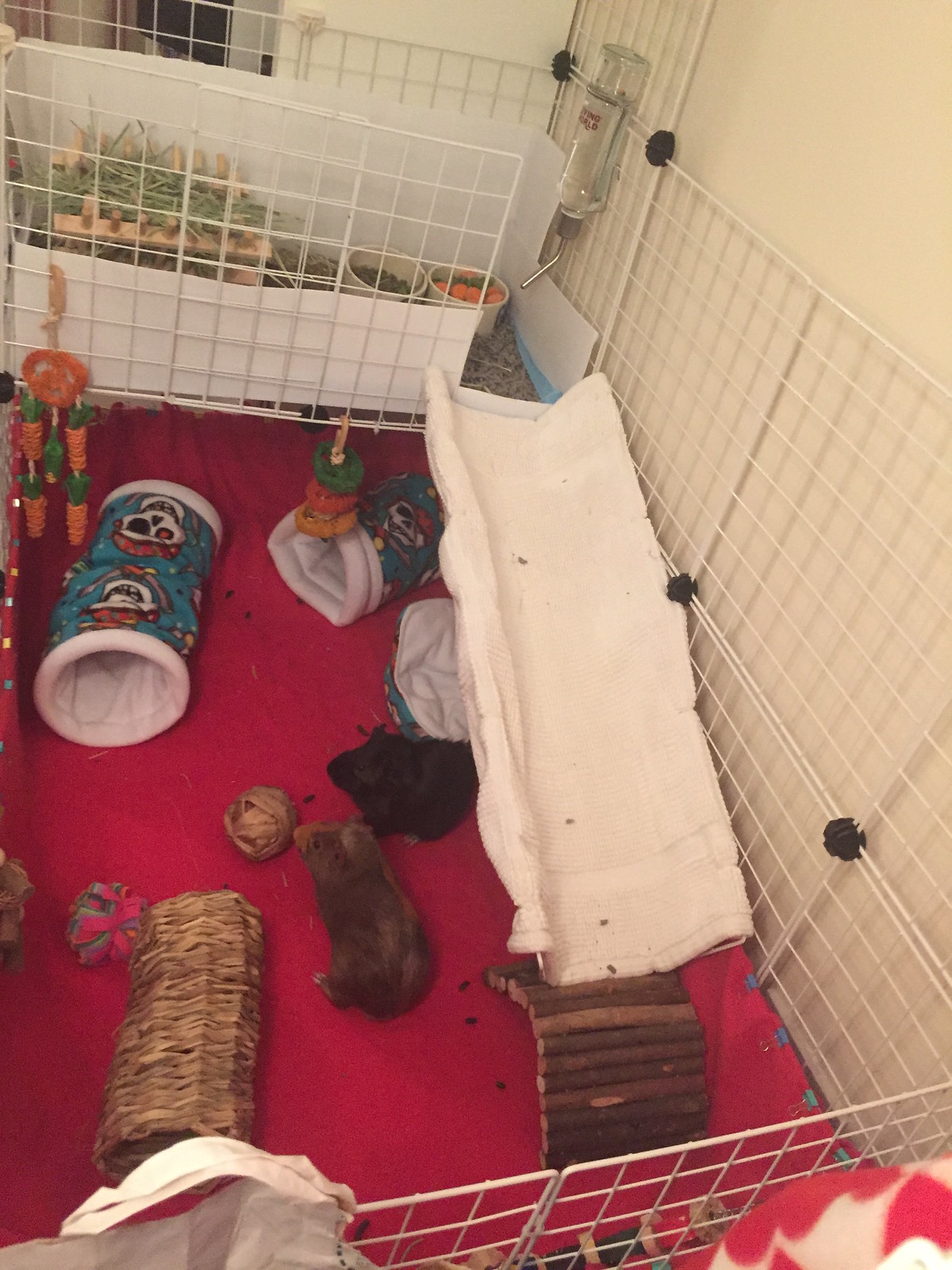An aerial view reveals a spacious, white guinea pig cage with open walls constructed from white metal fencing held together by black clips. The cage interior features a reddish-pink bottom mat and an array of playful accessories. Two guinea pigs inhabit the enclosure: one brown and facing away, the other black and looking to the right. Notable elements inside include a brown wicker tube and a distinctive white tube with a skeletal print on a blue background. At one end, there is a food tray accessible via a ramp that is covered in white material. Adjacent to the food tray, a water bottle hangs, and varied containers hold assorted foods, some of which are circular and possibly wooden. The setup is embellished with an abundance of toys and tunnels, including woven balls and tubes, ensuring an engaging environment for the guinea pigs. Numerous toys hang from the food tray, contributing to the rich variety of playthings in the enclosure.